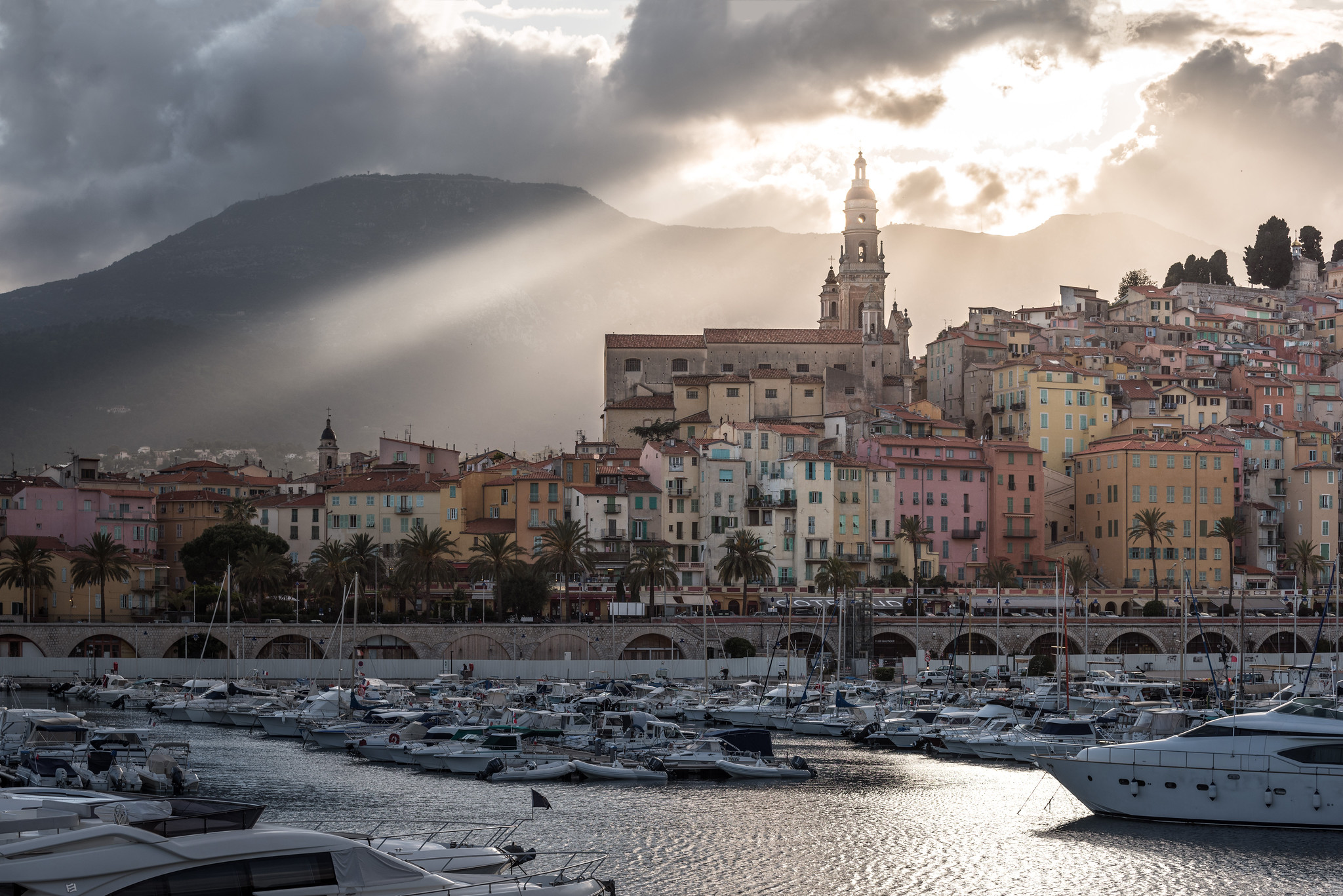This landscape-oriented photograph captures the charming coastal city of Menton, France. Taken from the harbor area, the bottom portion of the image is filled with numerous boats moored closely together on the serene water. Above the boats, a picturesque bridge with arches elegantly spans the scene, adding architectural interest. Higher up in the composition, an array of multi-level houses and large buildings, possibly apartments, climb the slope. Dominating the upper center to the right, a grand and impressive cathedral stands prominently. The backdrop features majestic mountains, partially veiled by clouds. The scene is bathed in the soft, golden hues of an impending sunset, with sun rays streaming beautifully across the sky. The light yellow coloration of the sunset adds warmth and tranquility to this idyllic snapshot of Menton's harbor at dusk.